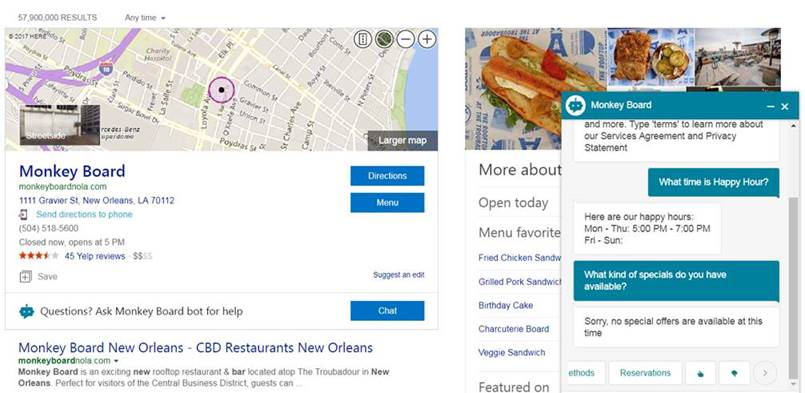**Detailed Caption:**

This screenshot from Bing Maps shows a detailed profile of the business, Monkey Board, located at 1111 Graveyard Street, New Orleans, Louisiana, 70112. The map section at the top of the screenshot features a prominent purple circle, indicating the business's location. A street-side photo insert occupies the lower left corner of the map, providing a visual representation of the area.

Below the map, the business information for Monkey Board is displayed. This includes the website (monkeyboardnola.com), address, and a contact phone number (504-518-5600). Monkey Board is rated 3.5 stars based on 4-5 Yelp reviews and is marked with 2 out of 4 dollar signs, indicating it is an affordable option. 

To the far right of the business information box, three blue buttons labeled "Directions", "Menu", and "Chat" provide quick access to respective functions.

Outside this main information box, a link and the title "Monkey Board, New Orleans, CDB Restaurant, New Orleans, monkeyboard.com" appear in green. To the right, another window is partially visible, indicating additional content related to the restaurant. This window features images of Monkey Board's food offerings and a pop-up chat window.

The chat window at the forefront shows an interaction between a customer and Monkey Board. The customer inquires about happy hour timings, to which Monkey Board responds that happy hour is from Monday to Thursday, 5 to 7 p.m., and there are no happy hour specials from Friday to Sunday. When asked about any current special offers, Monkey Board responds that no special offers are available at the moment. 

The chat interface includes a reservation option and thumbs-up/thumbs-down buttons for feedback. The customer's chat bubbles are teal, while Monkey Board's responses are in white.